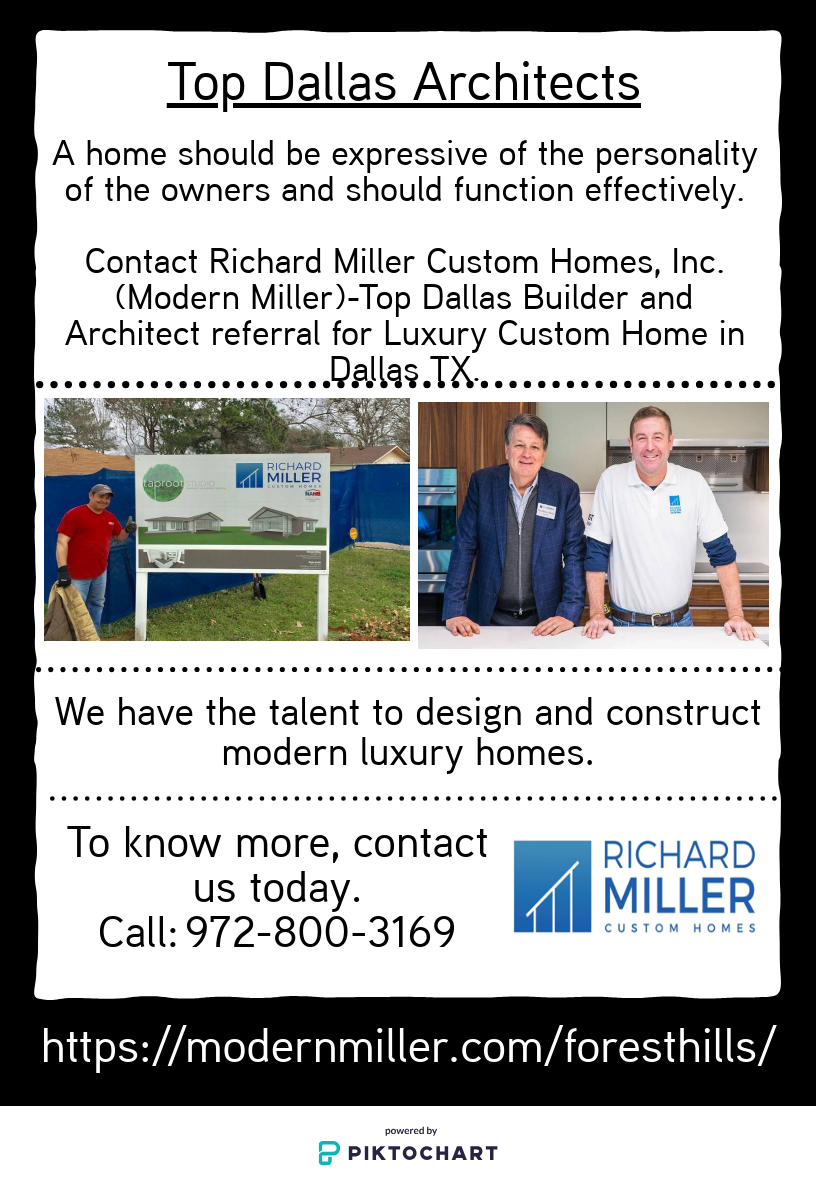This advertisement showcases the expertise of Richard Miller Custom Homes, promoting them as top architects in Dallas, Texas. It reads "Top Dallas Architects" at the top, followed by the statement: "A home should be expressive of the personality of the owners and should function effectively." It encourages potential clients to contact Richard Miller Custom Homes, a renowned builder and architect referral for luxury custom homes in Dallas.

The advertisement features two pictures: on the left, a person in a red t-shirt stands beside a Richard Miller sign in a residential yard, symbolizing successful project completions. On the right, two gentlemen, presumably the company's leading architects, are seen in a modern kitchen setting. One wears a blue jacket and the other a white jacket, both exuding professionalism and confidence.

At the bottom of the ad, there's a contact number, 972-800-3196, accompanied by the name Richard Miller and a blue square logo with a white railing, reading "Custom Homes." The website for further details is displayed in white letters against a black background.